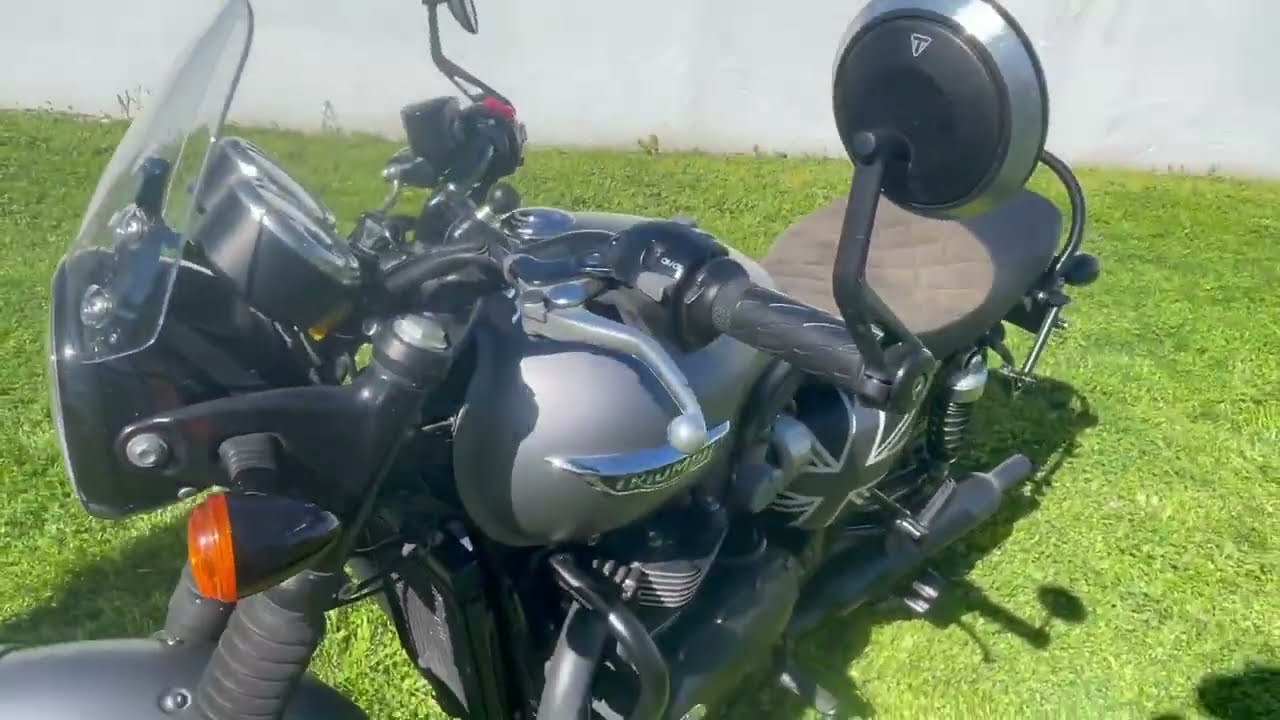This image depicts a high-end, premium sports motorcycle positioned on a verdant patch of green grass against a gray building wall. The motorcycle, predominantly gray and black, is a Triumph, as indicated by the brand name emblazoned on it. The visible design features include a large single headlamp, a small windshield, and exposed pipes, highlighting its classic yet modern aesthetic. Notably, there is an impression of a British flag in black and white under the seat. The photograph focuses on the intricately designed upper part of the bike, including the orange and black side light, while the tires are not visible. The backdrop is a simple gray wall, providing a stark contrast to the lush green grass below and emphasizing the sleek and sophisticated look of the motorcycle.